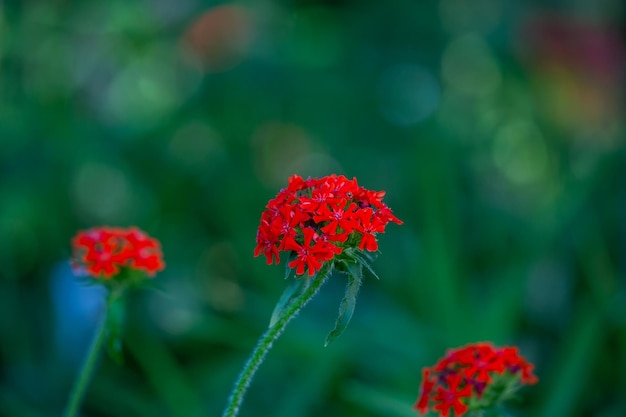This horizontal rectangular image showcases an intricate close-up of three bright red flowers, each crowning a green, hair-like spiked stem. The central flower, prominently positioned halfway up the image, is in sharp focus, revealing its numerous small, individual petals in a vibrant half-sphere shape. The flower is flanked by two long, thin leaves that drape gracefully downward. The two additional flowers, one on the left and one on the right, are slightly smaller and situated lower in the frame, resulting in a blur due to their distance and possibly their position nearer to the bottom edge. The entire composition is bathed in a vibrant green backdrop, which is heavily blurred, suggesting more plants or leaves, but with no distinct shapes, giving a bokeh effect reminiscent of a cloudy day with diffused lighting.